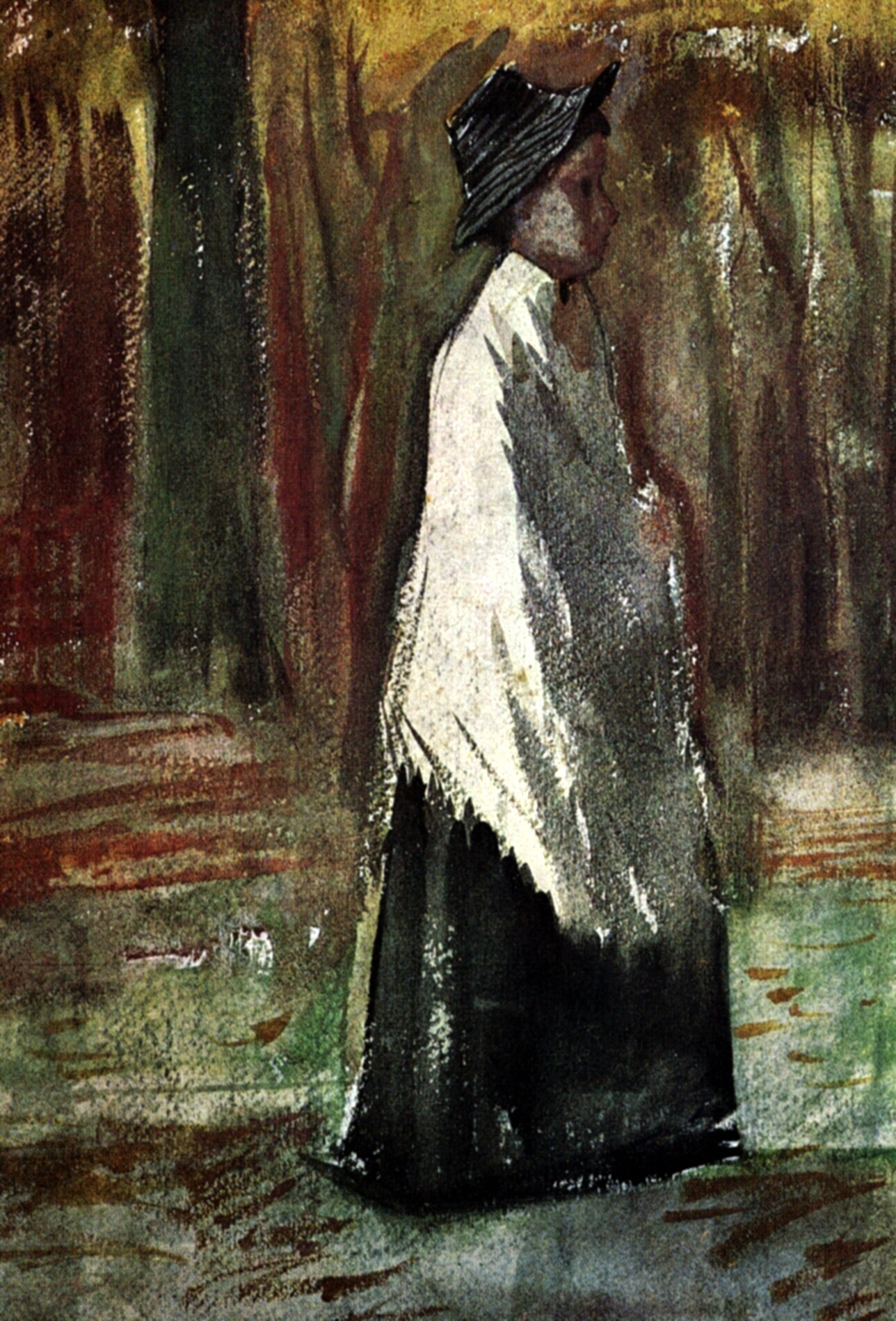The painting depicts an impressionist scene of a woman walking from left to right. She is adorned in a black hat and a distinctive outfit consisting of a long, white, mock cowl that nearly matches the length of her black dress which drapes down to her feet. The background suggests a natural, wooded setting with soft, vertical strokes of brown, yellow, and green that hint at trees and grass without providing clear detail. Additionally, there are deep red and green curtains depicted with vertical alignment and intersecting horizontal lines towards the center, adding to the painting’s abstract ambiance. The woman's gaze is directed to the right, peering off into the distance, enhancing the painting's somber and contemplative mood. The entire scene is rendered with impressionistic strokes, capturing the essence rather than the details of the subjects and environment.